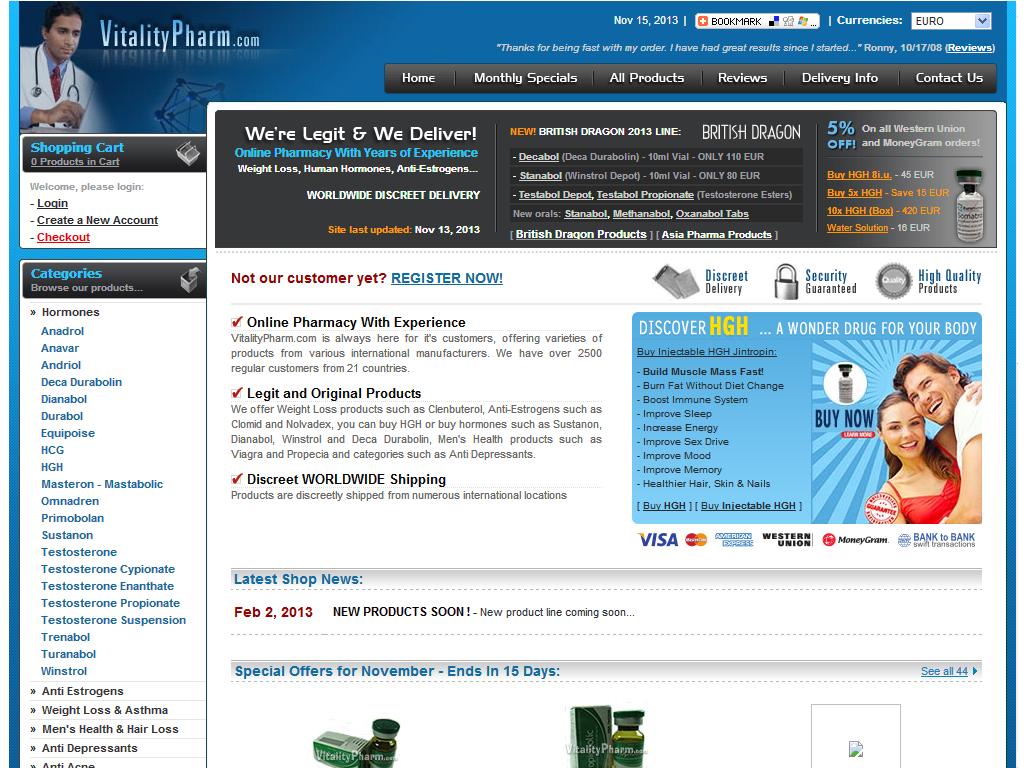This image is a detailed webpage snapshot from VitalityPharm.com, an online pharmacy specializing in various health products. 

In the upper left corner, a doctor is pictured with a stethoscope around his neck. He has dark hair and is looking towards the lower right corner, dressed in a blue shirt, red tie, and white lab coat. The background above him is a dark blue, with the website's name, "VitalityPharm.com," written in a lighter blue to the right of his head. The 'V' in Vitality and the 'P' in Pharm are capitalized. Adjacent to the website name are several white icons.

Further down and to the right of the doctor is a horizontal black section divided by thin vertical lines. The sections, labeled in white font, include: Home, Monthly Specials, All Products, Reviews, Delivery Info, and Contact Us.

On the left side of the page, there's a small vertical white rectangular area interrupted by a horizontal black section at the top that reads "Shopping Cart" in turquoise text. Below that, in gray text, it shows "Zero Products" and "Cart", accompanied by an icon. The subsequent section has a white background and gray text saying "Welcome, Please Log In." In bold black font below that, it says "Log In," followed by "Create a New Account," and "Checkout" in red. The section continues with "Categories" in turquoise text against a small black horizontal background. Below that, "Browse Products" is written in gray, and a column of product names follows. The first product, "Hormones," is in black font, and the subsequent names are in turquoise, including Anadrol, Anavar, Andriol, Deca, Durabolin, Dianabol, Durabot, Equipoise, HCG, HGH, Masterson, Mastabolic, Omadren, Premobolin, Sustanon, Testosterone, Testosterone Cypionate, among others, extending downwards.

The main body of the page is predominantly white, with a black horizontal stripe at the top displaying "We're Legit and We Deliver" in white font. Beneath it, in turquoise, the text reads "Online Pharmacy with Years of Experience." Additional details in white text read "Weight Loss, Human Hormones, Anti-Estrogen, Worldwide Secret Delivery," followed by more information.

Underneath, a bolded red text asks, "Not Our Customer Yet?" next to a turquoise "Register Now" in all caps. To the right, three icons with adjacent text highlight "Discrete Delivery," "Security Guaranteed," and "High Quality Products," with each phrase spanning two lines. The top words are turquoise, and the bottom words are black.

Three informational blurbs are present, each titled in bold black font with a red checkmark to the left. The titles are: "Online Pharmacy with Experience," "Legit and Original Products," and "Discrete Worldwide Shipping," each accompanied by further text.

On the far right, a turquoise or light blue section in all caps proclaims "Discover HGH," with "HGH" highlighted in yellow. Below this, in black font, is a list. The next section proclaims "A Wonder Drug for Your Body," featuring an image of a man and a woman with their arms around each other. In black font, it encourages "Buy Now," with additional details at the bottom.